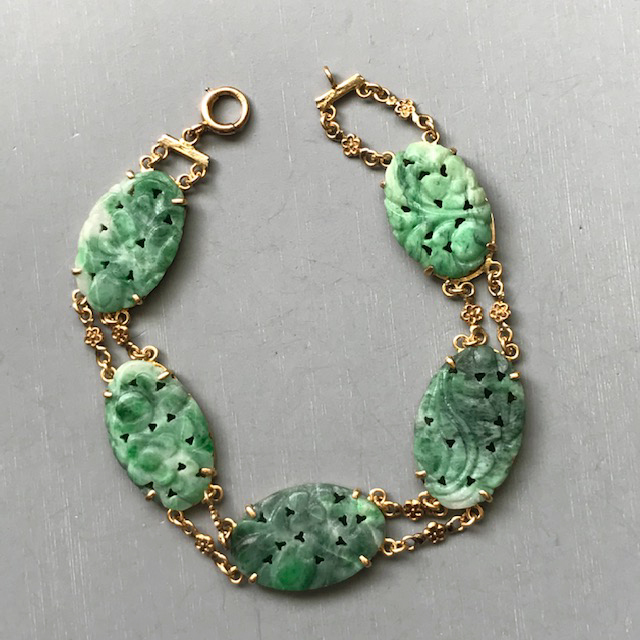Resting on a light gray surface, this detailed photograph captures an exquisite, vintage gold bracelet, likely of significant age and value. Centrally positioned in the image, the bracelet is unclasped, showcasing its intricate design. Made of double-link gold chains, it features five oval green gemstones, each varying in hues from almost white to dark forest green. These gemstones, possibly jade, are artistically adorned with tiny star, heart, or triangular cutouts, approximately eight per pendant, giving a decorative touch. The gemstones are connected in a linear sequence by two gold chain strings interlinking each gem. The bracelet is finished with a gold clasp at one end, highlighting its elegant craftsmanship. The photograph captures the piece in all its opulence, suggesting it is not only a statement piece but also a historical artifact worthy of a museum display.